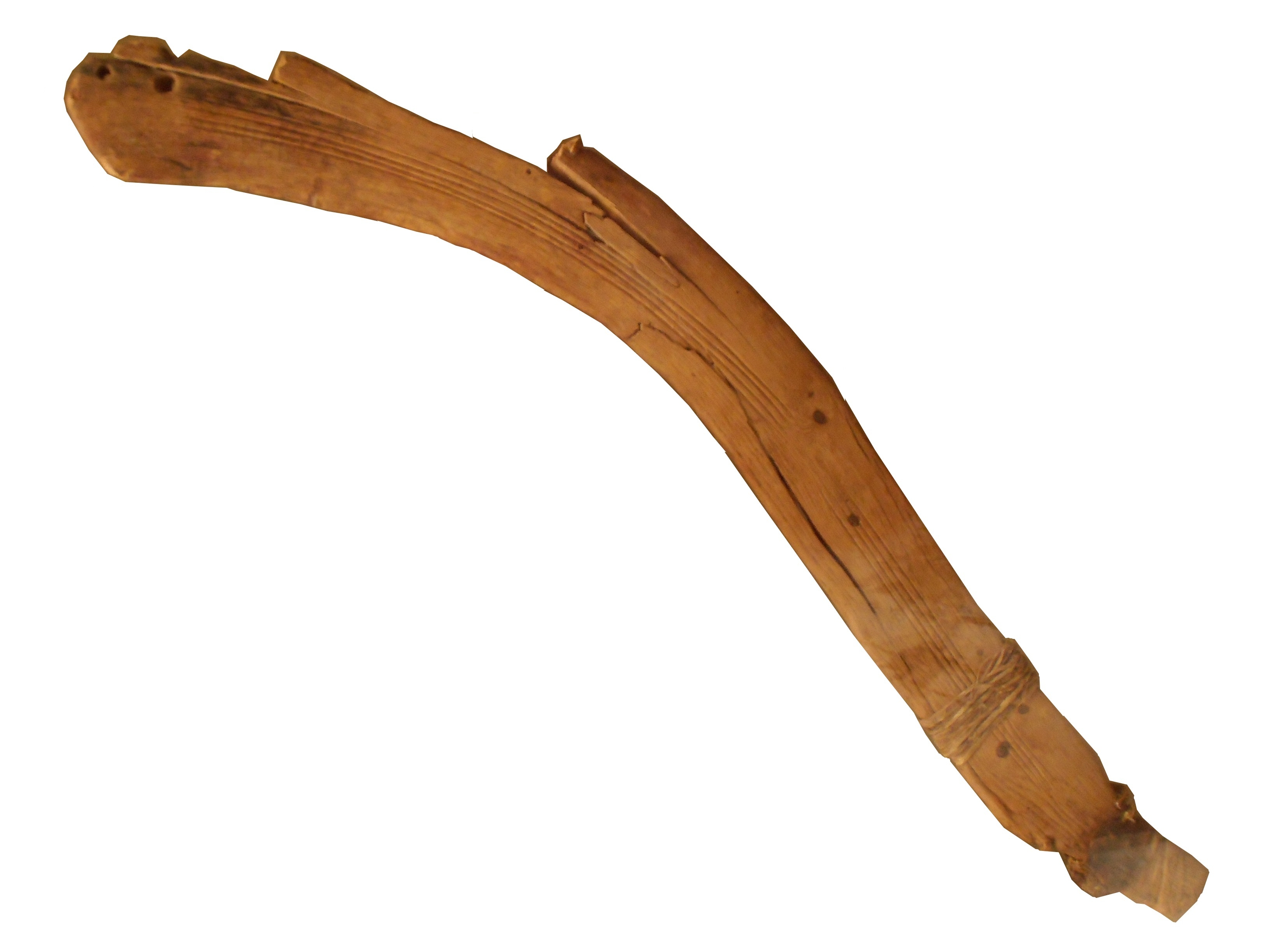The photograph presents a long and curved piece of wood set against a featureless white background that seamlessly blends with the frame, making the borders invisible. The wood seems to have undergone some form of carving, distinguished by striations along its length and several holes on its side, suggesting it might have been functional, possibly even a flute at one point. The artifact appears splintered at one end, though it's unclear whether this damage is recent or part of its original condition. The piece has a straight shaft that curves subtly to the left and features detailed carvings near one end, resembling the texture of rope. There's a small indention running along the bottom, culminating in a squared-off point at one end. The top edge shows wing-like protrusions, adding to its intricate design. Given its shape and craftsmanship, it might be a ceremonial object or an ancient tool, potentially hinting at cultural artifacts from regions like Australia or New Zealand. Its form brings to mind a boomerang, although its curvature is less pronounced than that of modern boomerangs. Overall, this carefully carved piece of wood suggests a purpose beyond that of a simple stick, enriched by cultural and functional significance.